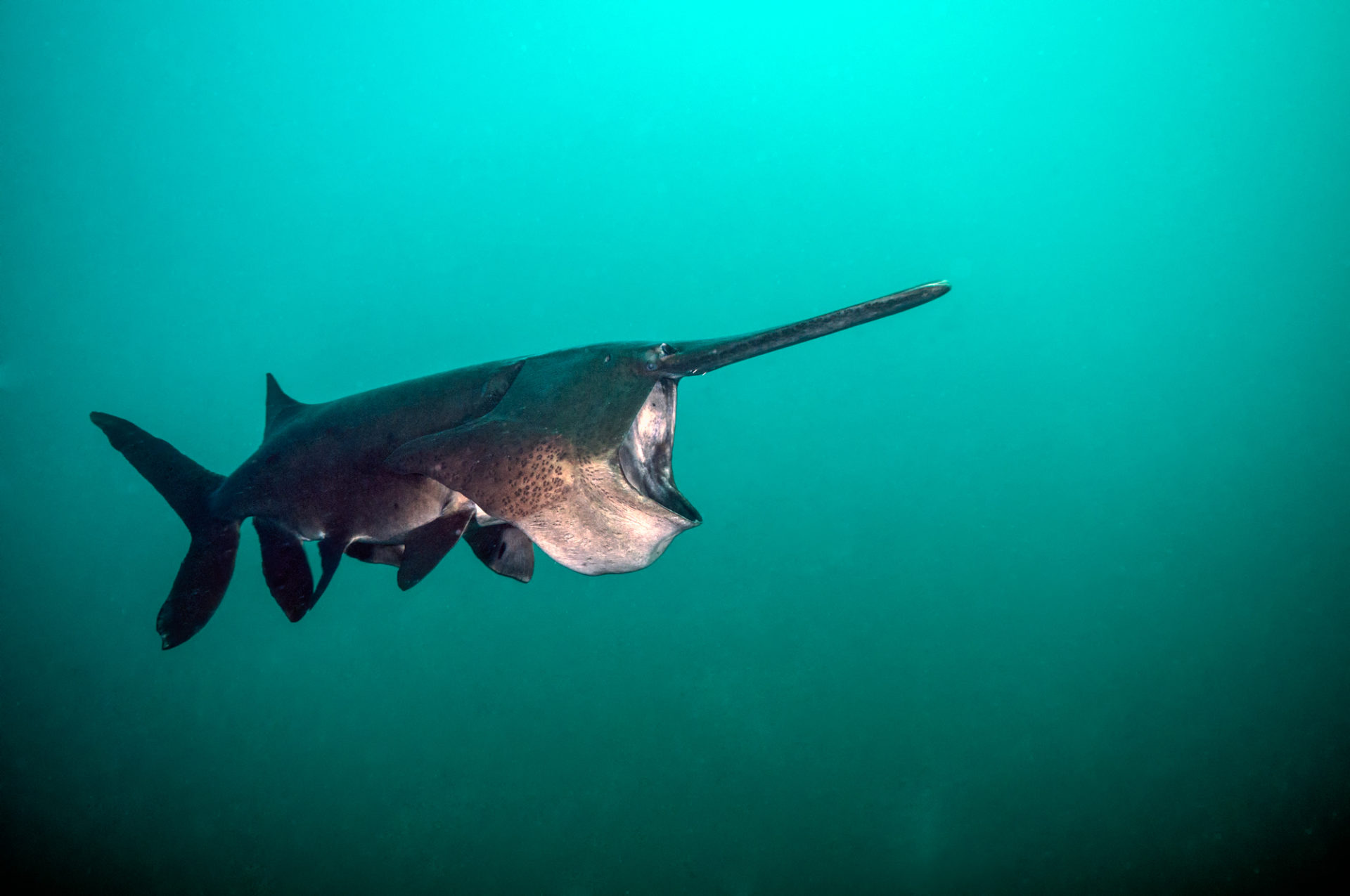This underwater photograph captures a fascinating, solitary fish or shark amidst a strikingly deep, greenish-blue background. The fish, positioned centrally and swimming from left to right, features a long, spear-like snout reminiscent of a swordfish. Its large, gaping mouth and spotted fins are distinctive, and its body exhibits a silvery, brownish-gray coloration. The water appears thick, hinting at the depth of the setting, with darker patches in the bottom corners adding contrast. The scene is both serene and captivating, emphasizing the isolated fish with its large jaws and strong, elongated tail gracefully cutting through the vibrant, clear waters.